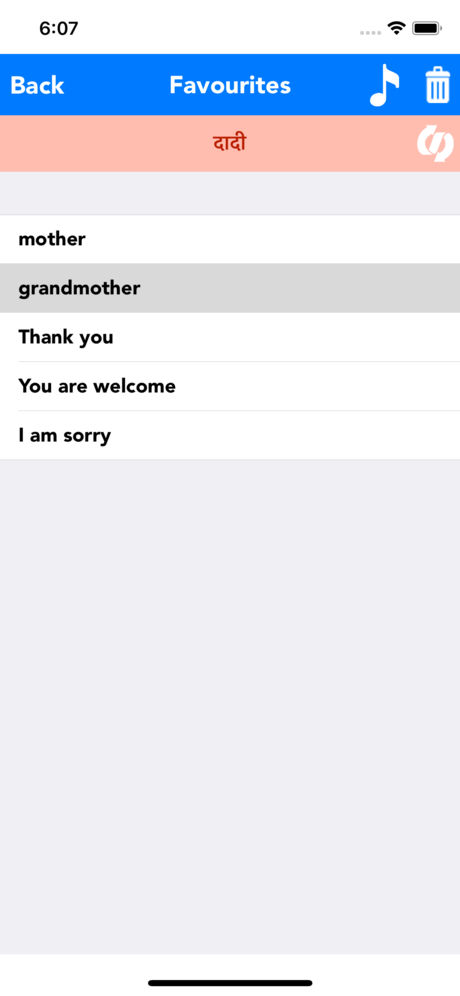The cell phone screen displays a detailed interface, starting with the status bar at the top left showing the time "6:07" and, on the right, icons indicating full cellular signal, active Wi-Fi connection, and a fully charged battery. Directly below this is a navigation bar colored in blue and white, with "Back" on the left, "Favorites" in the center, and icons for a music note and a trash can on the right side.

Moving further down, there's a peach-colored bar, prominently featuring text that appears to be in Sanskrit script, rendered in a rusty tan hue. Adjacent to the Sanskrit text on the right is an icon resembling the letter "S" formed by arrows, suggestive of a twisted ribbon. Below this, a thin gray band stretches across the width of the screen.

The main listing occupies the central portion of the display, comprising names such as "mother," "grandmother," "thank you," "you're welcome," and "I'm sorry." Each name is set against a white background, separated by fine gray lines. Notably, the entry for "grandmother" appears on a gray-highlighted band, distinguishing it from the others. 

Underneath the list, a larger light gray field is present, suggesting an area for additional content or input, punctuated only by a single black line centered within the space. Overall, the interface features predominantly black and white text, with the distinctive rusty color applied to the Sanskrit script, creating a visually organized, though somewhat cryptic, presentation that might relate to categorized favorites or commonly used phrases.